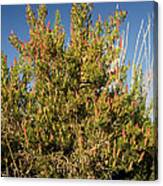The image showcases a small, low-resolution close-up of a blurry bush or shrub. The bush, which takes up most of the frame, has predominantly green leaves that appear yellow-green where the sunlight hits them. The foliage has hints of red at the top, adding an accent of color. Extending to the right side are some bare, whitish-yellow stems, indicating possibly dead parts of the plant. The bottom of the bush looks darker with visible small brown stalks, suggesting shadows or thicker areas of foliage. The background is a clear blue sky with some cloud cover near the lower part of the image. The plant seems untrimmed, growing irregularly in different directions, and hints at an arid environment, possibly surviving with minimal water.